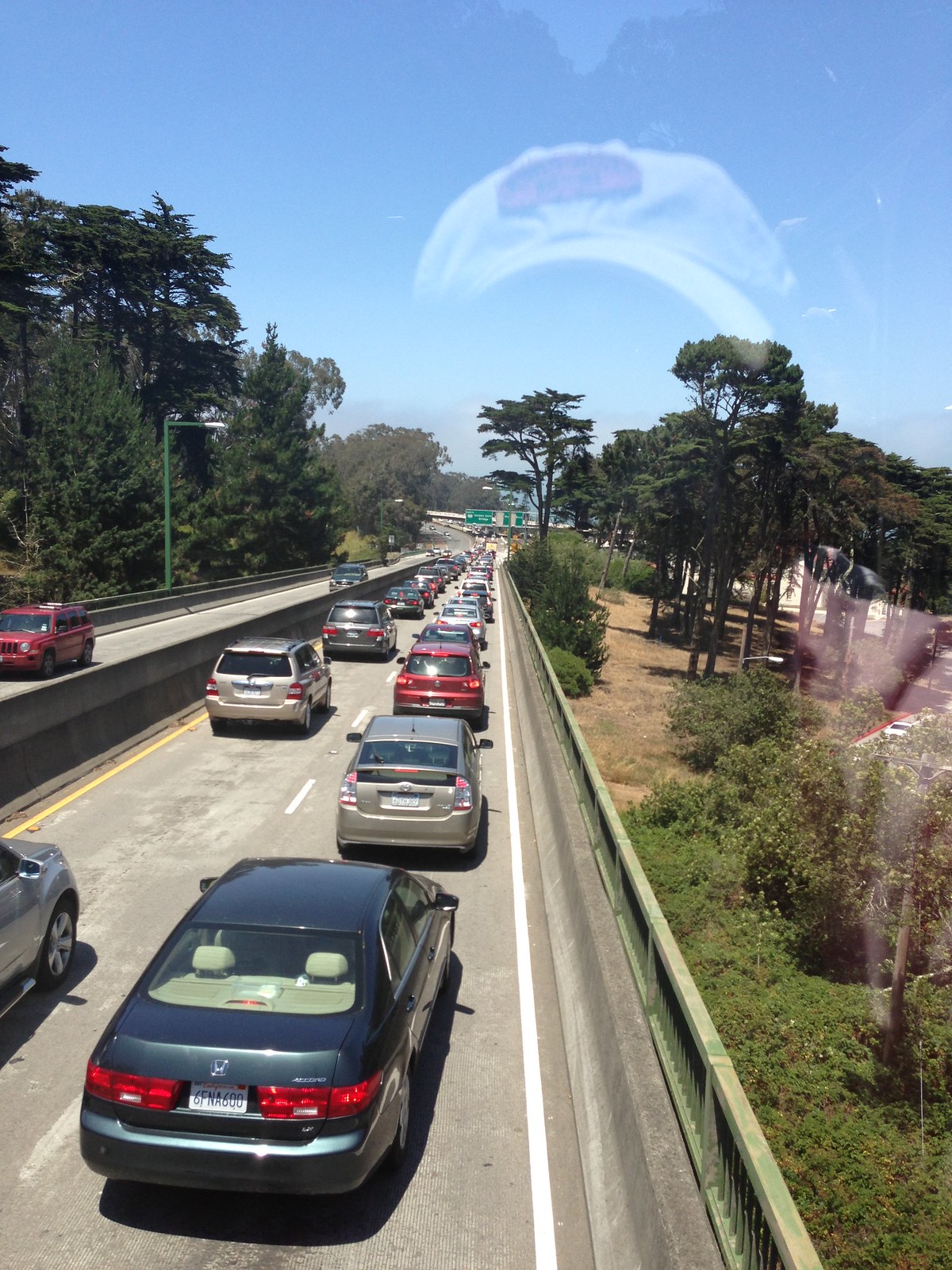The image captures a stretch of a California highway laden with backed-up traffic, specifically taken from atop a bridge with glass protection, as evidenced by the reflection of the photographer wearing a white hat. The highway has two lanes each for opposing directions - the far lane shows an unending line of vehicles moving away from the camera, while the nearer lane, directed towards the camera, is noticeably clear. Among the congested vehicles, a black sedan, a gray Prius, a red SUV, and a silver SUV are distinctively visible. The landscape flanking the highway features tall green trees and patches of grass, with a notable streetlight on a green post visible on one side. The scene extends endlessly under a light blue sky.